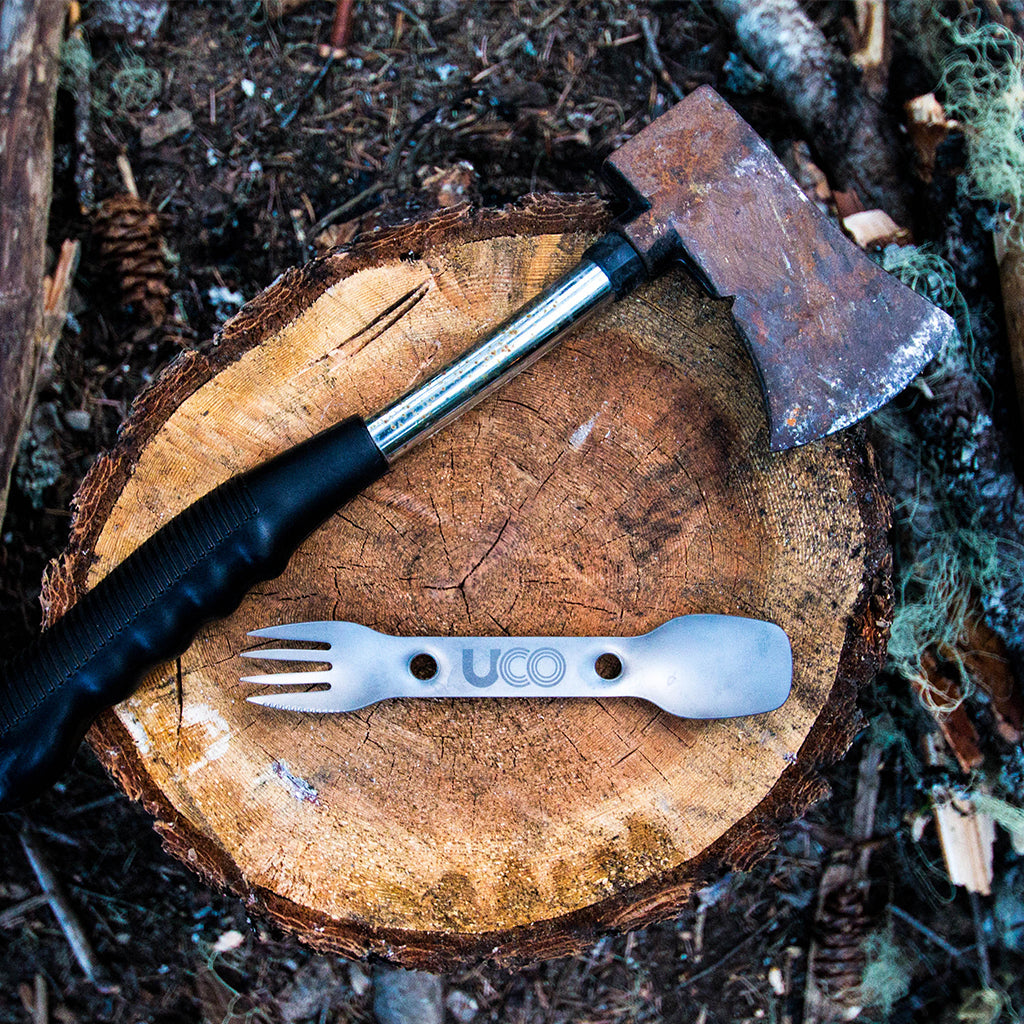This color photograph, framed in a square format, captures a slightly top-down view of a cut tree trunk placed on a forest floor, littered with dirt, branches, and scattered moss. The trunk, brown with visible grains, serves as a rustic backdrop for two camping items positioned on top. Near the upper left of the trunk, there's a weathered hatchet with a black plastic handle featuring a grip - its metallic neck transitions to a rusted iron head, angled such that the blade is at the top right corner and the handle extends to the bottom left. Below the hatchet lies a silver metal spork, with its forked prongs facing left and the spoon end to the right, connected by a central rectangular piece. Notably, the spork bears the inscription "UCO" in dark gray, stylish all caps lettering. The items rest in a natural setting, enhancing the scene's realistic, representational photographic style.